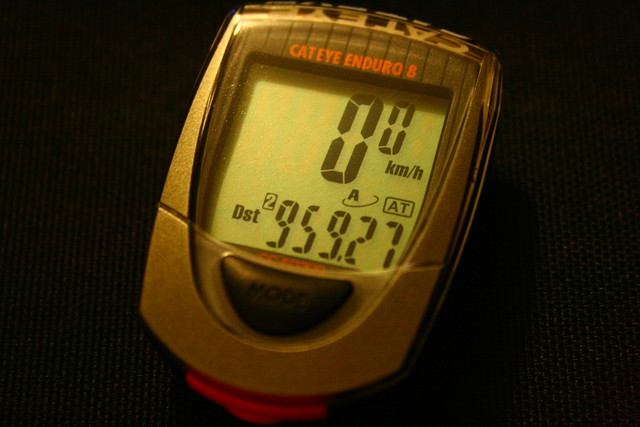The image features a square-shaped timer, predominantly gold or a light silver color, made of plastic. At the top of the timer, the brand name "CATEYE" and the model name "ENDURO 8" are prominently displayed in red. The device has a digital screen situated below these inscriptions. The digital display shows a large zero, a smaller zero on the right side, and the units "KM/H" underneath the zero. An assortment of other labels and numbers is visible on the screen, including "DST," the number "2," a small black square, and the sequence "959.27". Between the zeros and "959.27," there's a small "A" encircled by an arrow. Within the small black square, the letters "AT" are inscribed. Below the digital screen is a semi-circular black button with the word "MODE" engraved on it in white letters. The bottom edge of the timer features a hint of red coloring. The device is lying on a black surface, providing a stark contrast that makes the details of the timer more prominent. The word "CATEYE" is also inscribed in white capital letters at the very top edge of the timer.